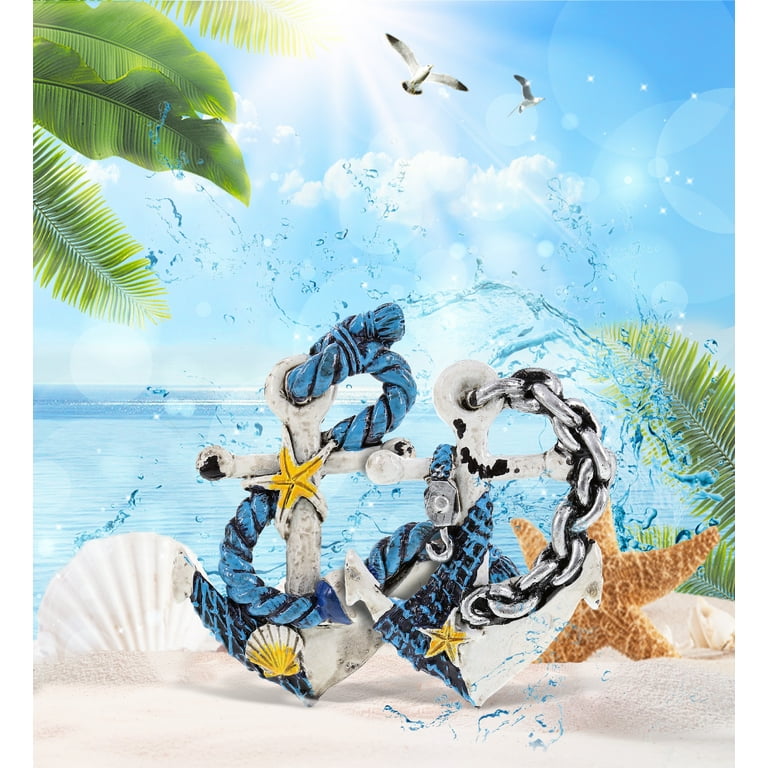This image is an advertisement for coastal wall decor, featuring a beautiful beach scene. The backdrop showcases a vivid blue sky with sunlight streaming down from the top center, casting a radiant glow. Puffy clouds dot the sky, while flecks and beams of sunlight enhance the scene's brightness. In the top left corner, palm leaves gently frame the view, and two seagulls soar gracefully across the sky. The sandy foreground is adorned with various seaside elements: green palm leaves, a big splash of water, and three distinct shells—one is white, another is tan, and the third is a seashell. Central to the composition are two T-shaped anchors, designed with a blend of materials such as cast resin, metal, or concrete, and painted in shades of blue and yellow. The anchors are entwined with ropes or metal chains, featuring a netting texture. Both anchors are decorated with starfish and seashells, enhancing the coastal theme. The detailed elements and vibrant hues create a harmonious and tranquil beachside atmosphere, perfect for wall decor.